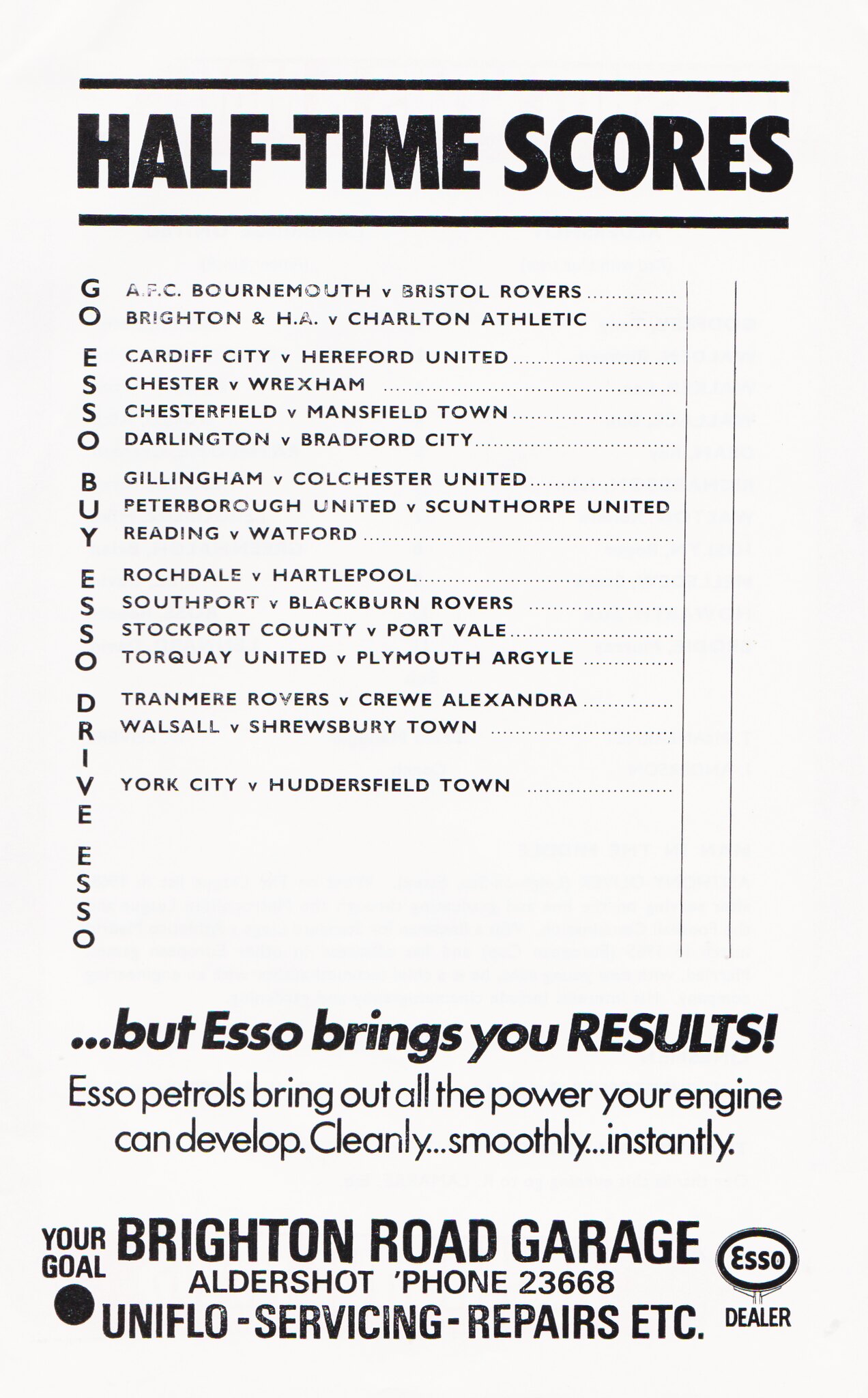The image appears to be a scanned, vintage newspaper or magazine page that predominantly features an advertisement for Brighton Road Garage. The page is headed with the bold, capitalized, sans-serif text "HALF-TIME SCORES," which is both underscored and overscored by thick black lines. Below this heading, several pairs of team names are listed, such as "APC Bournemouth" vs. "Bristol Rovers" and "Brighton" vs. "Charlton Affleck," with adjacent columns likely intended for score entries. Notably, the left side of the page has vertical text saying "Go SO, Buy SO, Drive SO." At the bottom, an advertisement is prominently displayed, emphasizing SO petrols with the bold assertion, "but SO brings you results!" and detailing how "SO Petrols bring out all the power your engine can develop cleanly... smoothly... instantly." The ad also includes contact information for Brighton Road Garage in Aldershot, directing readers to phone 23668, and ends with mention of "Uniflow servicing, repairs, etc." The background of the entire page is white, ensuring the black text and details stand out clearly.